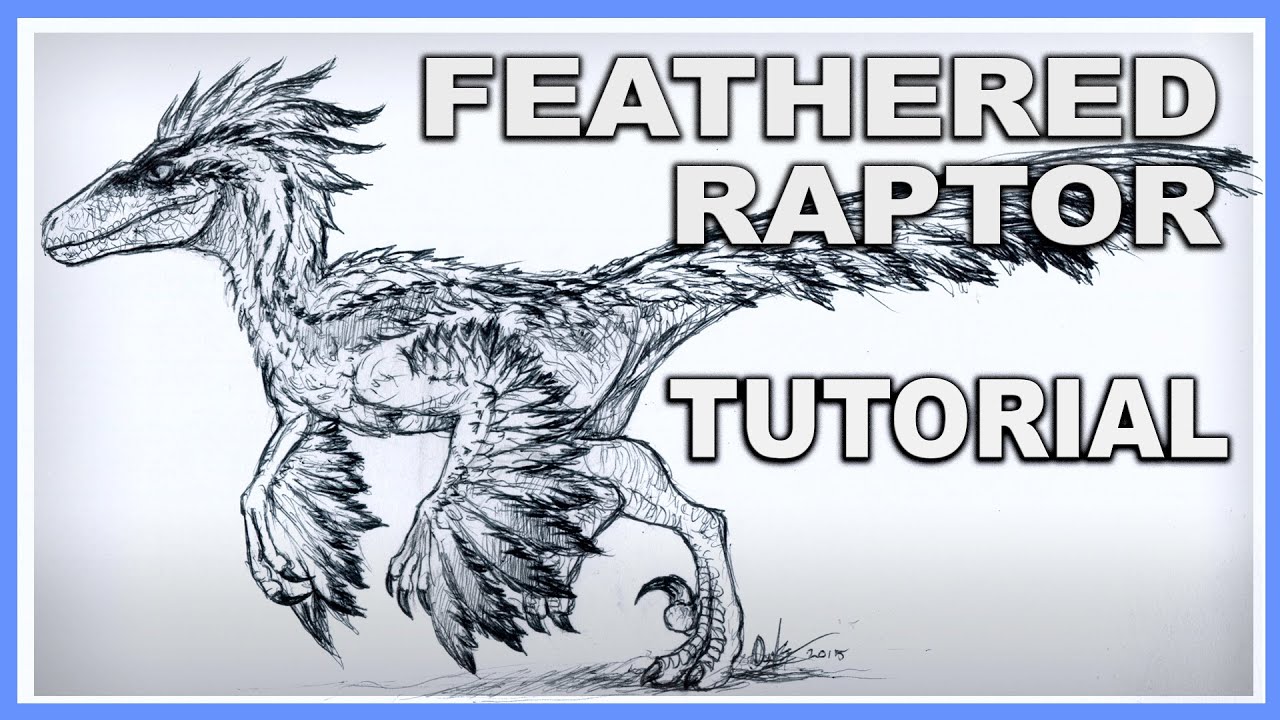The image is a horizontally aligned rectangle with a medium blue border. Inside the border, the background is a light gray color. In the center is a black-and-white sketch of a dinosaur running towards the left, resembling a Velociraptor with prominent feathers on its head, arms, and tail, giving it a bird-like appearance. The dinosaur's head is on the left side of the image, and its tail extends to the right. Overlaid on the upper right side and extending towards the center are the words "FEATHERED RAPTOR" in large block letters, outlined in black, with the word "TUTORIAL" underneath. This text is right-aligned and is so large that it spans into the middle of the image. The overall composition suggests it could be a cover or thumbnail for a video, clearly highlighting the theme of the Feathered Raptor Tutorial.